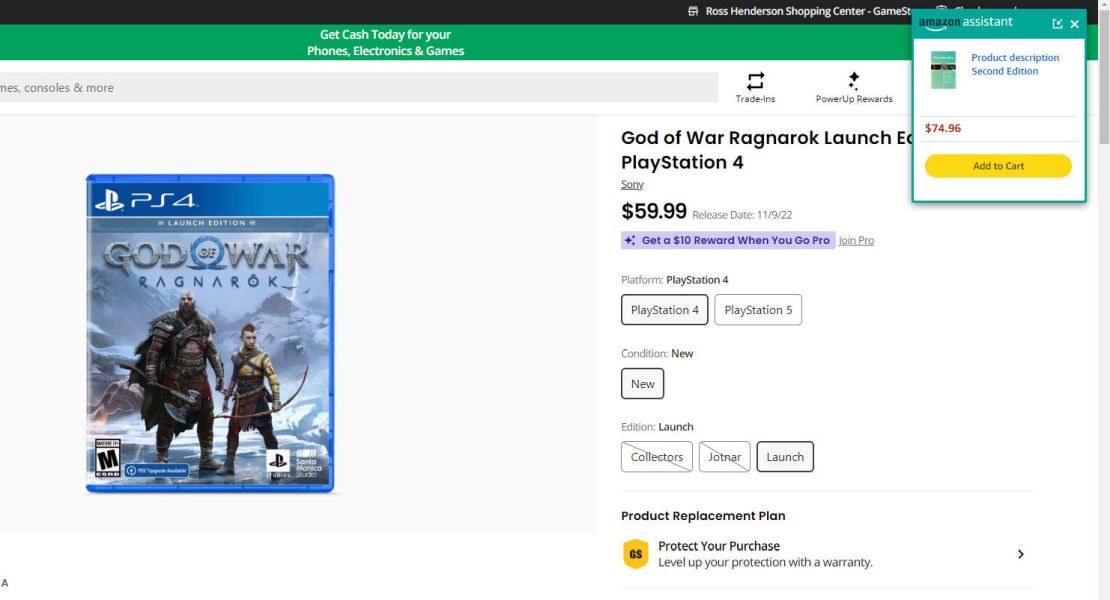This image captures the purchase page for "God of War Ragnarok" on the PlayStation 4, likely hosted on a video game retail site similar to GameStop. The central feature is an image of the game's front cover, depicting an older warrior, wielding a formidable axe, positioned alongside a younger man armed with a bow and arrow. They stand against a backdrop of towering mountains, evoking an epic and adventurous atmosphere.

To the right of the game's cover image, there are options for selecting the gaming platform and the condition of the game. The top right of the page includes the presence of the Amazon Assistant, offering additional purchasing suggestions. The product is described as the second edition, priced at $74.96, with an "Add to Cart" button readily available for convenience.

Beneath the purchasing options, there is an offer to add a warranty to protect the purchase. The overall layout allows potential buyers to carefully view and evaluate the game, complete with the distinct blue PS4 case that houses the game disc.